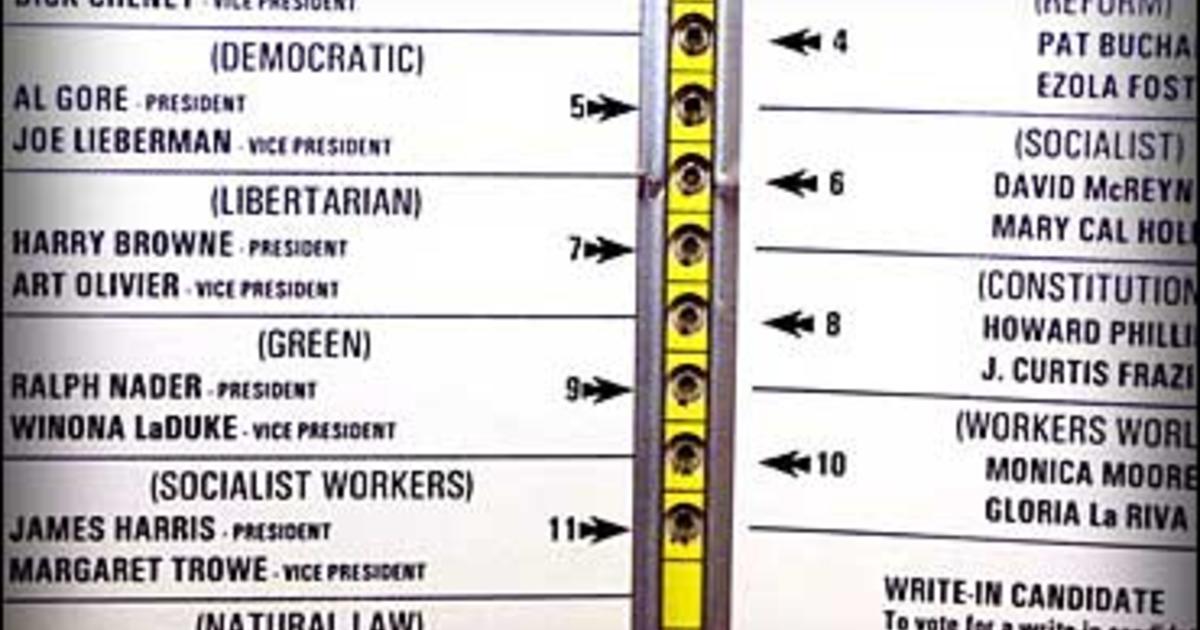This is a detailed, close-up view of a punch card ballot from the 2000 U.S. presidential election. The ballot features candidates from multiple parties, including Democrats Al Gore for President and Joe Lieberman for Vice President; Libertarians Harry Brown and Art Olivier; Green Party candidates Ralph Nader and Winona LaDuke; and Socialist Workers candidates James Harris and Margaret Trow. The image captures a portion of the ballot where other candidates, such as those from the Reform, Socialist, Constitution, and Workers World parties, are partially visible but their names are cut off. Notably, there's also a section for write-in candidates. The punch card holes are prominently placed in the center, allowing voters to punch their selection. The image underscores the complex and potentially confusing layout of the Florida ballots, which was a significant issue during the 2000 election. A yellow strip with punch card dots runs down the middle of the ballot, highlighting the physical interaction required to cast a vote.